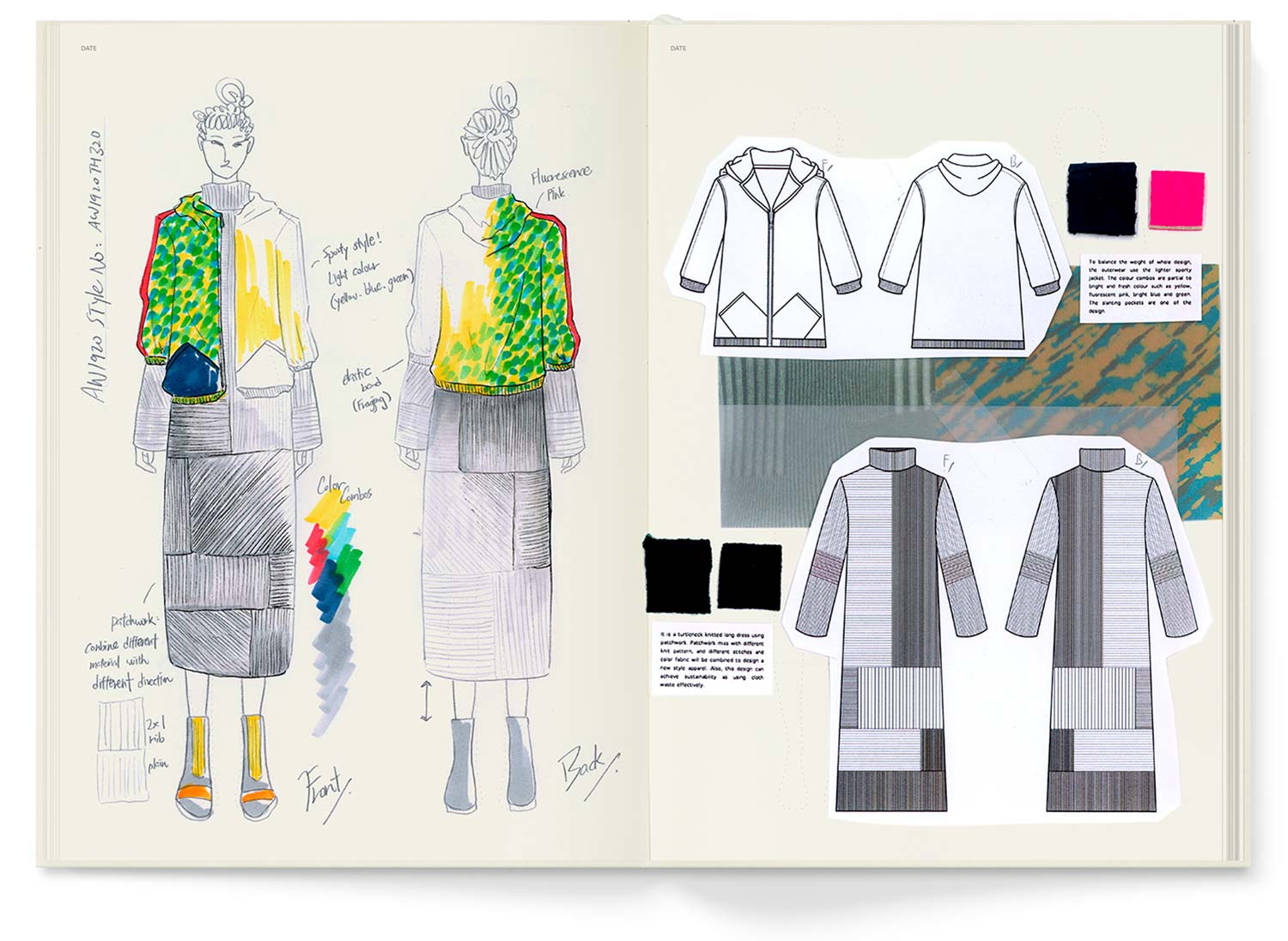The image displays a highly detailed fashion design reference for a woman's clothing, primarily in black and white with selective color highlights. On the left side, the front view illustration of a woman features a striking jacket with yellow on one side and green and yellow on the other, adorned with a blue pocket on the left. The design includes red stripes and green dots on a yellow background, complemented by vertical and slanted lines. The woman, who has curly hair and a turtleneck, also wears boots with yellow and orange stripes.

Adjacent to this front view is the back view of the same woman, showcasing the rear details of the jacket. This depiction maintains the green and yellow elements with a red stripe and green dots continuing around the back. Notably, her boots lack the color details seen in the front view.

To the right of these figures, there are two more jacket designs, each accompanied by squares indicating color swatches and fabric patterns. These squares feature different textures and colors, including black, pink, and tan-blue camouflage, along with black and gray fabrics with stripe patterns.

Additional text annotations around the images provide material and style information, albeit difficult to read. These annotations likely indicate details about the fabrics and stitching instructions. The overall drawing is meticulous, possibly derived from a fashion design book, detailing horizontal and vertical lines of fabric, various shading, and construction notes.